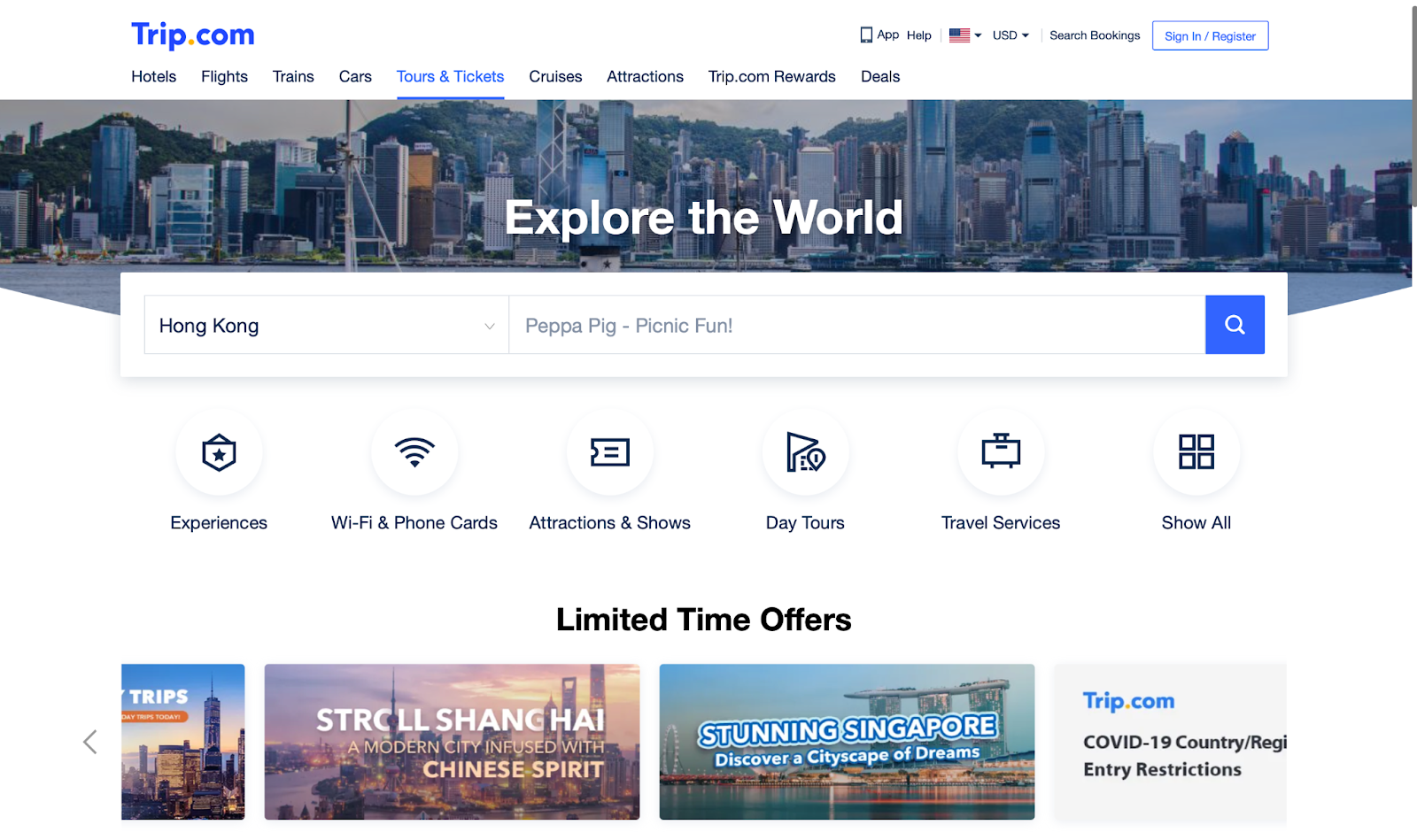"Trip.com Landing Page

The landing page of the Trip.com website prominently displays the title 'Trip.com' in the upper left-hand corner. Dominating the page is a captivating image of a dense urban city skyline, which is not clearly identifiable as an American city. Overlaying this cityscape is the headline 'Explore the World,' set in bold typography. Beneath this headline, a search box displays the dropdown selection 'Hong Kong,' though it's unclear if Hong Kong is the actual city pictured.

Adjacent to the search box is another input field featuring the placeholder text 'Peppa Pig Picnic Fun' in grey, suggesting a common search term but not currently active. Directly below these search features are six icons, each representing different categories: 'Experiences,' 'Wi-Fi and Phone Cards,' 'Attractions and Shows,' 'Day Tours,' 'Travel Services,' and 'Show All.'

Further down the page, a section labeled 'Limited Time Offers' features a series of engaging images leading to other destinations. One image, overlaid with the text 'STRCLL Shanghai, a modern city infused with Chinese spirit,' presumably depicts a scene from Shanghai. Another image titled 'Stunning Singapore, Discover a Cityscape of Dreams' seemingly represents Singapore. Additionally, there is an important icon labeled 'Trip.com COVID-19 Country Register Entry Restrictions,' providing vital information for travelers regarding travel restrictions.

This highly visual and user-friendly layout aims to entice visitors to explore various travel options and services offered by Trip.com."